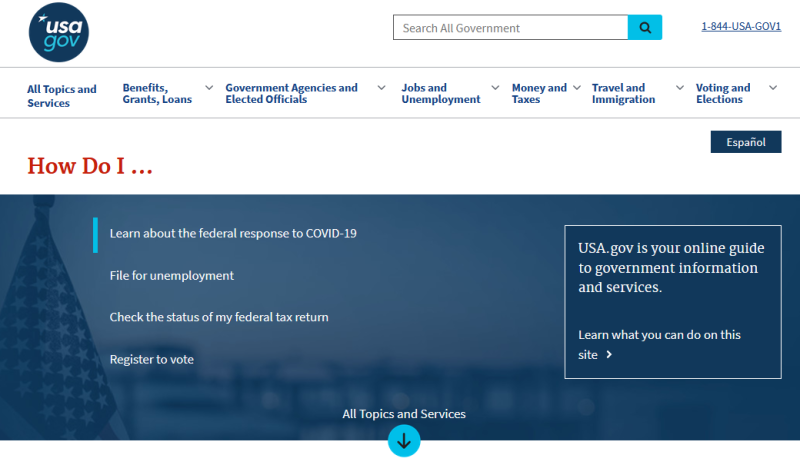This is a detailed screenshot of the USA.gov website. At the very top, there is a white menu bar featuring a search bar on the left and the USA.gov logo in the top left corner. The logo consists of a dark blue circle with "USA" in white lettering and "GOV" in light blue below it. The search bar is equipped with a blue search button on its right side, and further to the right is a phone number, displayed as a blue link: 1-844-USA-GOV-1.

Below the search bar, there is a horizontal navigation menu containing seven blue links aligned across the top. To the right of this menu, there's a dark blue "Español" button. Directly below the navigation menu, on the far left side, is an orange highlighted section titled "How do I..." with trailing ellipses. At the very bottom of the screenshot, there is a section with a blue background.